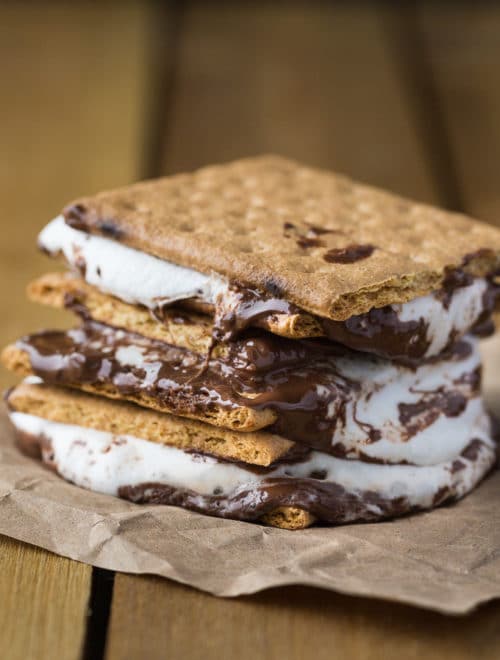A delectable close-up image features a sumptuous dessert snack crafted from square-shaped graham cookies. These cookies, exhibiting a slightly dark golden brown hue and characteristic hole-punched tops, are stacked in a tempting tower. Sandwiched between the layers of cookies, luscious melted chocolate and gooey marshmallows ooze and drip enticingly, cascading down the sides and pooling at the edges to create a mouth-watering visual delight. The entire confection rests atop a piece of brown paper, which in turn is set on a light, dull brown wooden table, adding a rustic charm to the overall presentation.